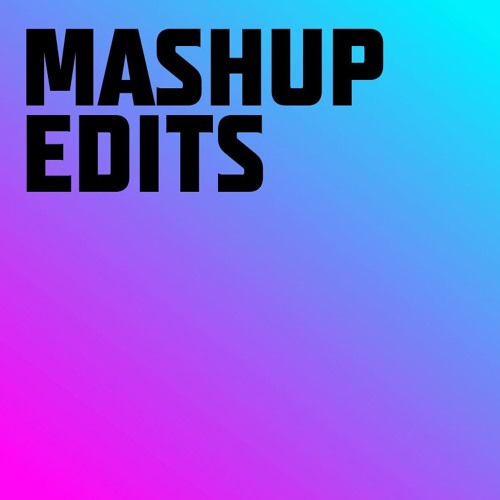The image is a simplistic square design reminiscent of album art, characterized by a gradient effect that transitions diagonally. Beginning from the top right corner, the gradient starts as a light blue, gradually shifting to a medium blue, then a darker blue, and finally fading into purple and pink in the bottom left corner. Positioned in the top left of the image, slightly staggered to the left, is the bold, black text "Mashup Edits" written in all capital letters, with "Mashup" on the top line and "Edits" just below. The overall design lacks other distinguishing features, emphasizing its basic yet striking gradient effect and prominent text.